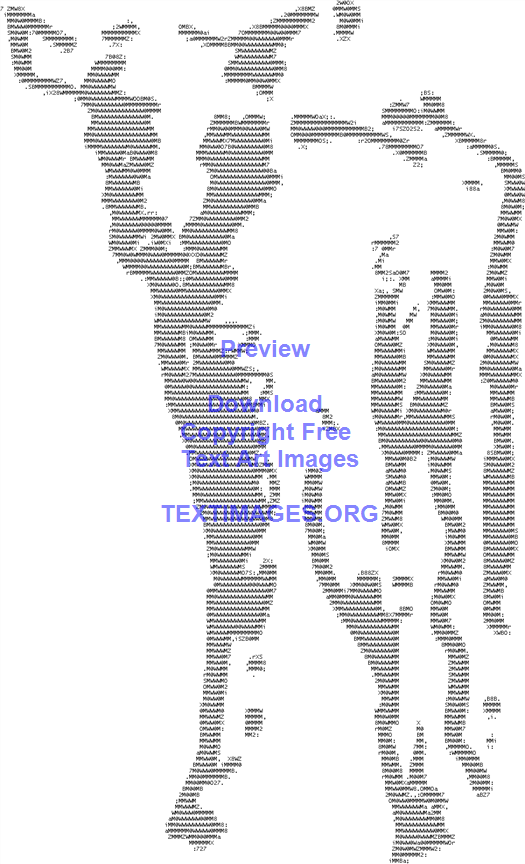The image is a computer-generated, black-and-white pixelated silhouette of a calf facing forward and slightly to the left. The silhouette is detailed with various keyboard characters forming the outline, depicting its ears, eyes, nose, legs, and body. A distinct white streak runs down just to the right side center of its face, while most of its body remains white except for some black lines along its left side from its leg up to its head. In the center of the image, the word "PREVIEW" is prominently displayed in blue letters, followed by "DOWNLOAD," "COPYRIGHT FREE," "TEXT ART IMAGES," and "TEXTIMAGES.ORG" at the bottom, all separated by spaces. These elements suggest a focus on text art images.